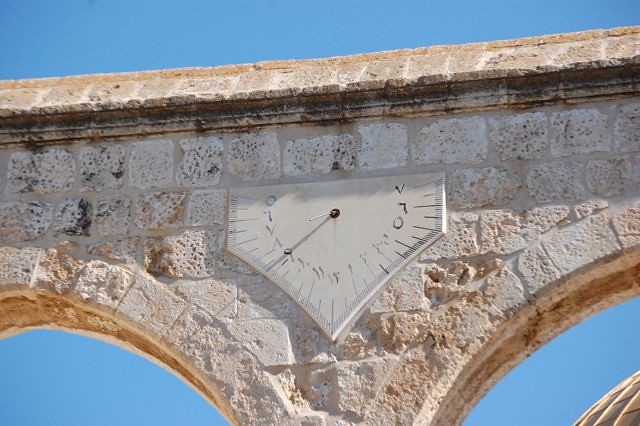In this image, we observe an intricately designed clock or meter, presumably intended for measuring some type of data. The numerals on this device are rendered in Arabic numerals, providing a universal sense of readability. This clock is mounted on the side of a substantial concrete structure, likely a bridge or an architectural archway.

The base of this structure is notable for its carved-out sections that form an arch shape, defining the architectural aesthetic. The top portion smooths out into a single, continuous panel that resembles a roof, providing a stable background for the clock face.

The clock design itself is curiously triangular and features a single prominent hand, possibly indicating time or some other measurement. There appears to be a secondary, smaller hand, but it is difficult to distinguish clearly due to pixelation. The overall image conveys an intriguing blend of functional engineering and architectural elegance.